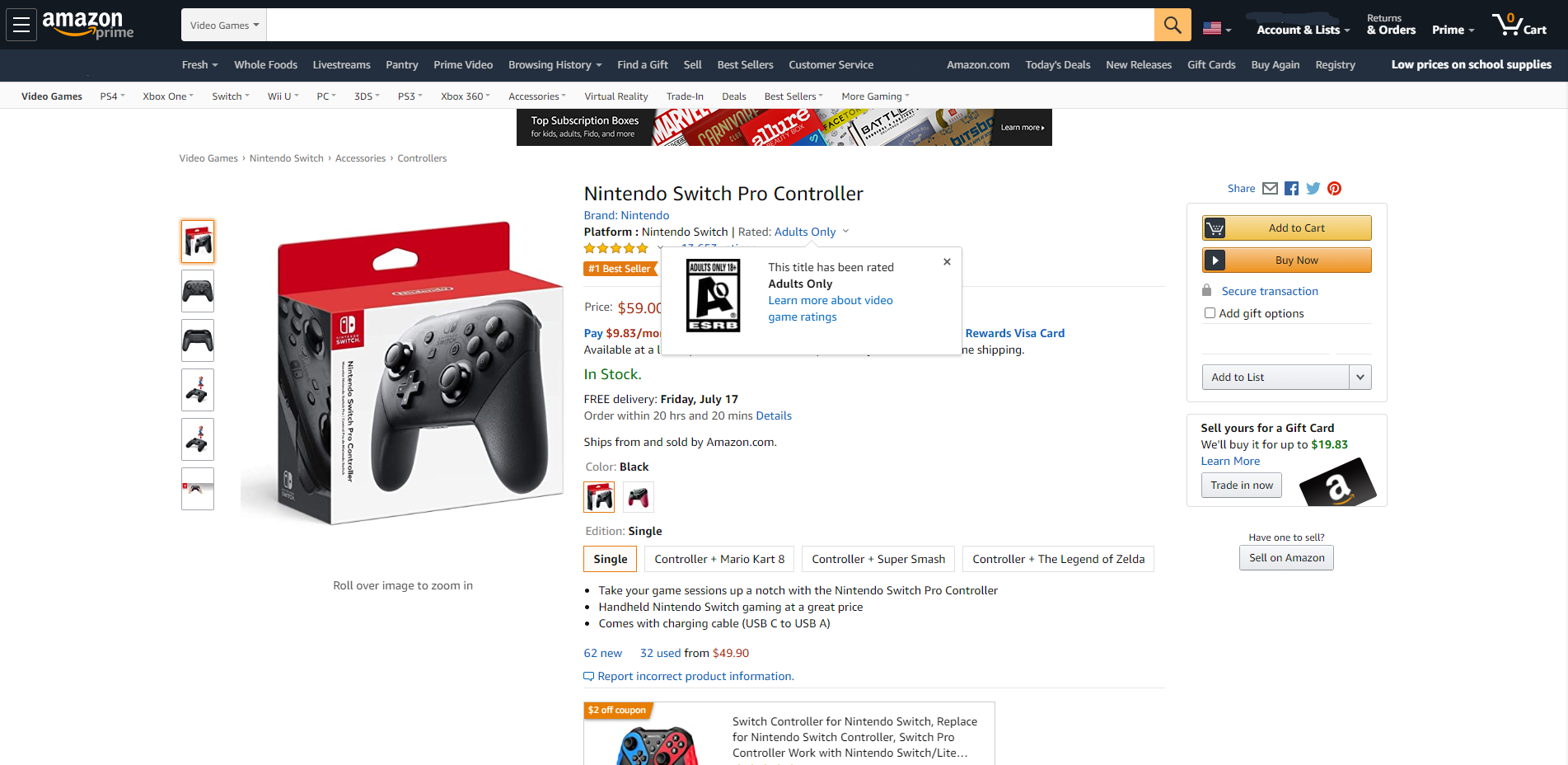This is a detailed caption for an image showing a color screenshot of an Amazon page:

"The screenshot displays an Amazon webpage featuring a black banner at the top. On the far left, the banner includes the Amazon Prime logo with an orange circle and an orange arrow connecting the 'A' to the 'Z' in the traditional Amazon logo. On the far right, the banner lists 'Account & Lists,' 'Returns & Orders,' 'Prime,' 'Zero,' and 'Cart.' Centered on the black banner is a search bar, set to the 'Video Games' category.

The item showcased is the 'Nintendo Switch Pro Controller,' under the brand 'Nintendo' for the 'Nintendo Switch' platform. It has a rating of 'Adults Only.' The user has clicked on 'Adults Only,' leading to a pop-up window informing that the title is rated 'Adults Only,' with a link to learn more about video game ratings. Adjacent to this pop-up on the left is a black and white box displaying 'Adults Only, 18+, AO, ESRB.'

To the left of this box is a photograph of the Nintendo Switch Pro Controller, which is black and depicted on the front of its packaging against a white background, with the top part of the box in red. Below the image, the price is listed as '$59,' with an installment option of 'paid $9.83/month' partially obscured by the pop-up about the Adults Only rating. The item is marked 'In stock,' offering 'Free delivery by Friday, July 17,' if ordered within '20 hours and 20 minutes.' Details note it 'Ships from and sold by Amazon.com,' with options for 'Color: Black' and 'Edition: Single.' Additional options include 'Single,' 'Controller + Mario Kart 8,' 'Controller + Super Smash,' and 'Controller + Legend of Zelda.' A promotional line states, 'Take your game sessions up a notch with the Nintendo Switch Pro Controller, handheld Nintendo Switch gaming at a great price. Comes with charging cable, USB-C to USB-A.'"